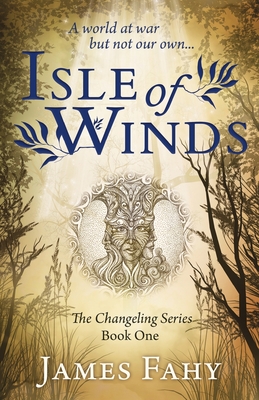This is an image of the front cover of the book "Isle of Winds" by James Fahey, part one of The Changeling series. The background of the cover is composed of sepia tones, including browns, beiges, and tan colors, giving it a vintage, rustic feel. Framing the edges are tall grass and trees, creating an impression of a forest. At the top, the heading in italicized sentence case reads, "A World at War, But Not Our Own." 

The title "Isle of Winds" is prominently displayed in a stylized blue font, with artistic branches bearing leaves extending from the 'W' and 'F.' Below the title, there is a central image of an ornate tree with extensive roots, which cleverly form a face. This artwork stands out against the earthy background, complemented by sunlight filtering through the tree canopy. Beneath this image, it is noted that this is Book One of the series, "The Changeling Series."